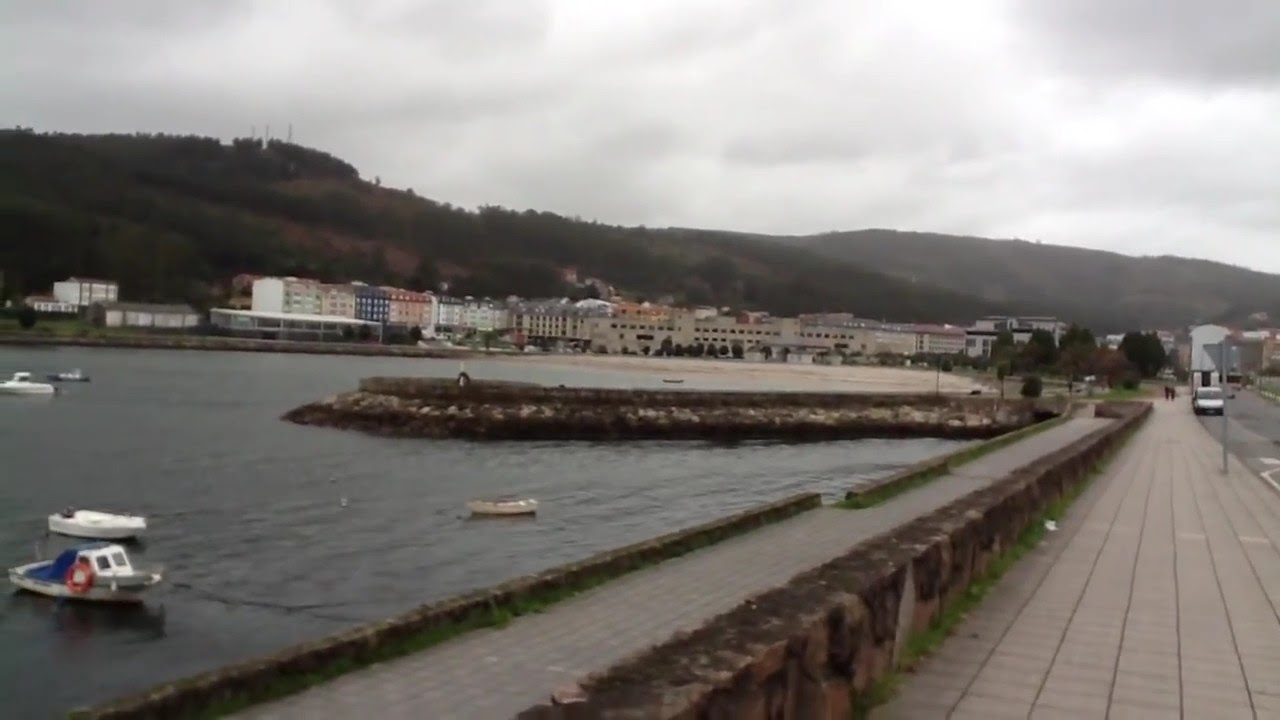The photograph captures a bustling bay area under a gray, cloudy sky during the daytime. Dominating the foreground is a large body of slightly rippled water, populated by several small, mostly white personal fishing boats. One notable boat features a buoy and a blue tarp at its rear. Adjacent to the water, on the right, lies a long, concrete and tiled walkway flanked by a retaining wall that doubles as a fishing spot. Beyond the walkway is a sidewalk, followed by a road lined with multiple parked cars and a distant vehicle, possibly a bus.

In the background, a sprawling array of connected buildings, varying in colors from beige to navy to light pink, stretches along the base of a green, tree-covered hillside. Dirt paths snake through the hilly landscape, which continues to the horizon, imparting a slightly mountainous feel. Off in the distance, the buildings rise to about three to five stories high, suggesting a mix of residential and commercial structures. The shoreline also features rocky formations and a grassy, tree-lined port area, adding depth and contrast to the scene. Small human figures can be spotted on the sidewalk, providing a sense of scale to this dynamic, scenic bay area.